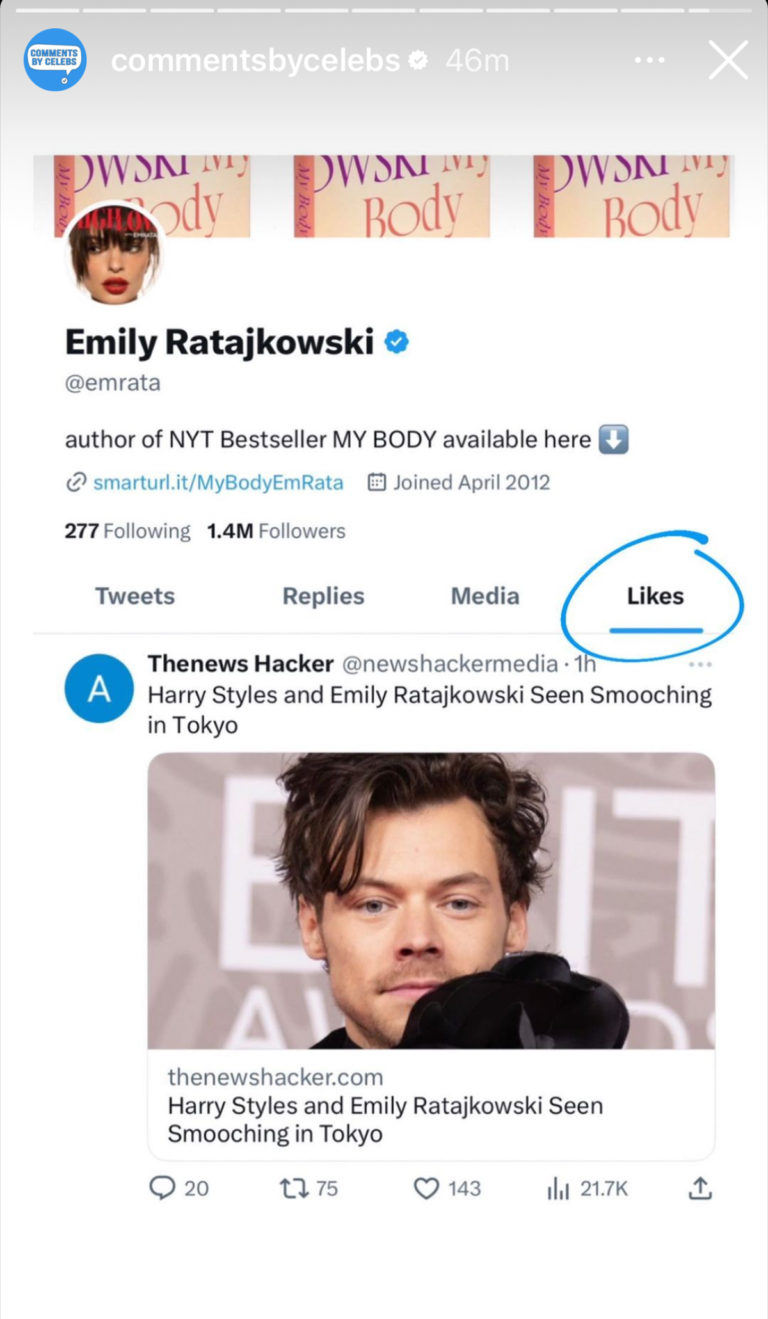Detailed screenshot of a social media app on a smartphone. At the top of the screen, there is a blue circle with the text "Comments by Celebs," followed by "Comments by Celebs" and a verified blue checkmark. The timestamp reads "46 minutes ago," with an ellipsis for more options and an 'X' button to close. Above this, several white bars indicate navigation through additional screens.

Below that, a user profile is displayed, featuring a screenshot prominently showcasing books related to the person. The central image captures a female face with red lipstick and brown hair, identified as Emily Ratajkowski, whose name is verified with a blue checkmark on Twitter under the handle @emrata. The profile description includes: "Author of NYT Bestseller, My Body, available here," followed by a link: smarturl.it/mybodyemrata. Emily joined Twitter in April 2012, is following 277 accounts, and has 1.4 million followers. Tabs for "Tweets," "Replies," "Media," and "Likes" are shown, with the "Likes" tab currently selected and underlined.

Below Emily's profile, a tweet from "The News Hacker" with the handle @newshackermedia, posted one hour ago, is visible. The post reads: "Harry Styles and Emily Ratajkowski seen smooching in Tokyo," accompanied by a picture of Harry Styles.